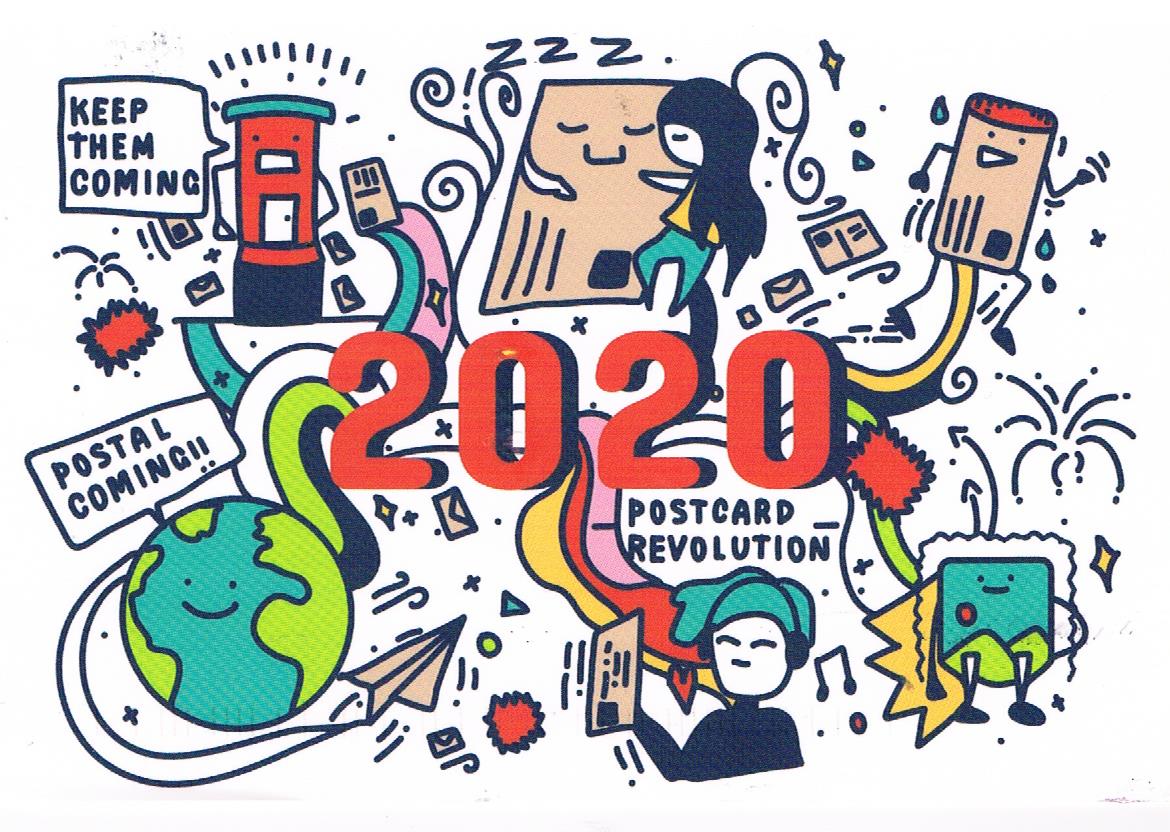The image features a collage on a white background, combining hand-drawn elements and colorful clip art. Central to the composition is "2020" written in large, medium red letters with a black shadow on the right side, giving it a 3D effect. Directly beneath "2020," in uppercase black letters, the phrase "POSTCARD REVOLUTION" stands out. Scattered around the central text are various symbols and illustrations related to postcards and mailing. These include:

- A building in the upper left corner with the phrase "KEEP THEM COMING."
- A symbol of the Earth and the phrase "POSTAL COMING" in the lower left.
- In the upper right, a paper airplane and a letter with legs are depicted running.
- Toward the center, a letter with a ZZZZ above it, indicating sleep.
- A smiling girl holding a letter.

The artwork captures numerous themes related to postcards and mailing, using a mix of whimsical and expressive visuals to reflect the concept of a postcard revolution in the year 2020.